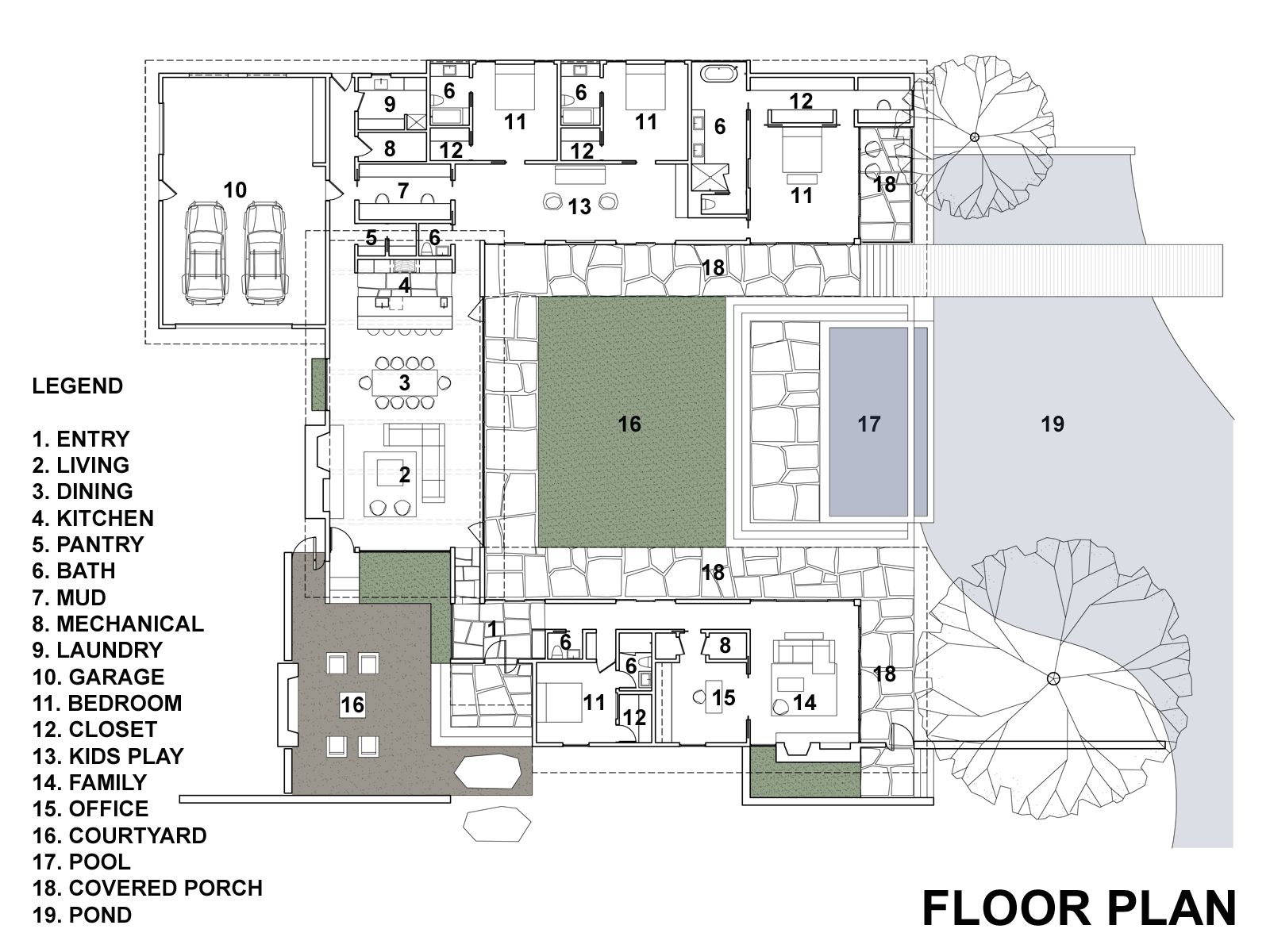This image depicts a detailed blueprint of a house floor plan, labeled with "floor plan" in bold black letters at the bottom right. The layout outlined in the blueprint includes 19 numbered areas, identified in a legend located about halfway up the left side. The legend details include: 1. Entry, 2. Living, 3. Dining, 4. Kitchen, 5. Pantry, 6. Bath, 7. Mud, 8. Mechanical, 9. Laundry, 10. Garage, 11. Bedroom, 12. Closet, 13. Kids Play, 14. Family, 15. Office, 16. Courtyard, 17. Pool, 18. Covered Porch, and 19. Pond.

The blueprint is mainly in black and white, with certain sections highlighted in shades of green and gray for clarity. The courtyard (16) is shaded green, while the pool (17) features a dark grayish blue, and the pond (19) is a lighter gray. The main portion of the layout shows the boundaries and markings of all rooms and features, with specific notes such as a two-car garage in the upper left, a pool near the center right, adjacent to a pond, and the main courtyard area positioned at the center and lower left of the blueprint. The overall design showcases a comprehensive view of the house from above, indicating it is a residential structure, complete with family-oriented spaces like a family room and a kids' play area.